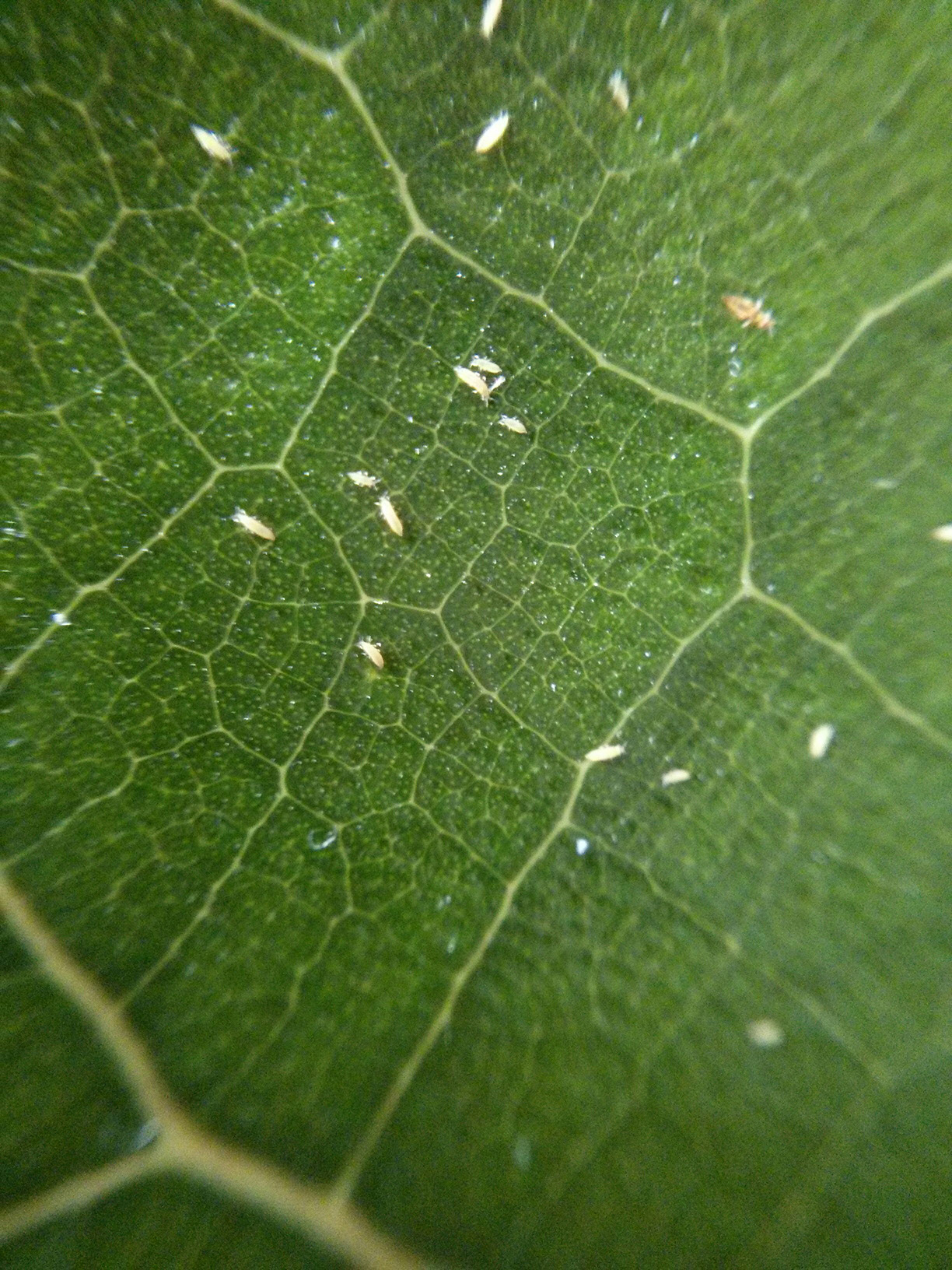This close-up photograph of a green leaf showcases the detailed texture and structure of its surface, emphasizing the intricate network of raised veins. These veins create a delicate pattern of smaller cells within the leaf, characteristic of its vascular system, and appear in lighter shades of green and white. The rich green color of the leaf suggests it is healthy and abundant in chlorophyll, the pigment responsible for photosynthesis. Scattered across the surface are tiny white specks, which might be dust, fungal spores, or pest eggs. Among these specks, there are also small white and slightly larger brown bugs, possibly aphids, with visible legs. The white bugs resemble grains of rice, while the brown ones are slightly more defined. Tiny water droplets glisten on the leaf, adding to the detailed texture captured in this photograph.